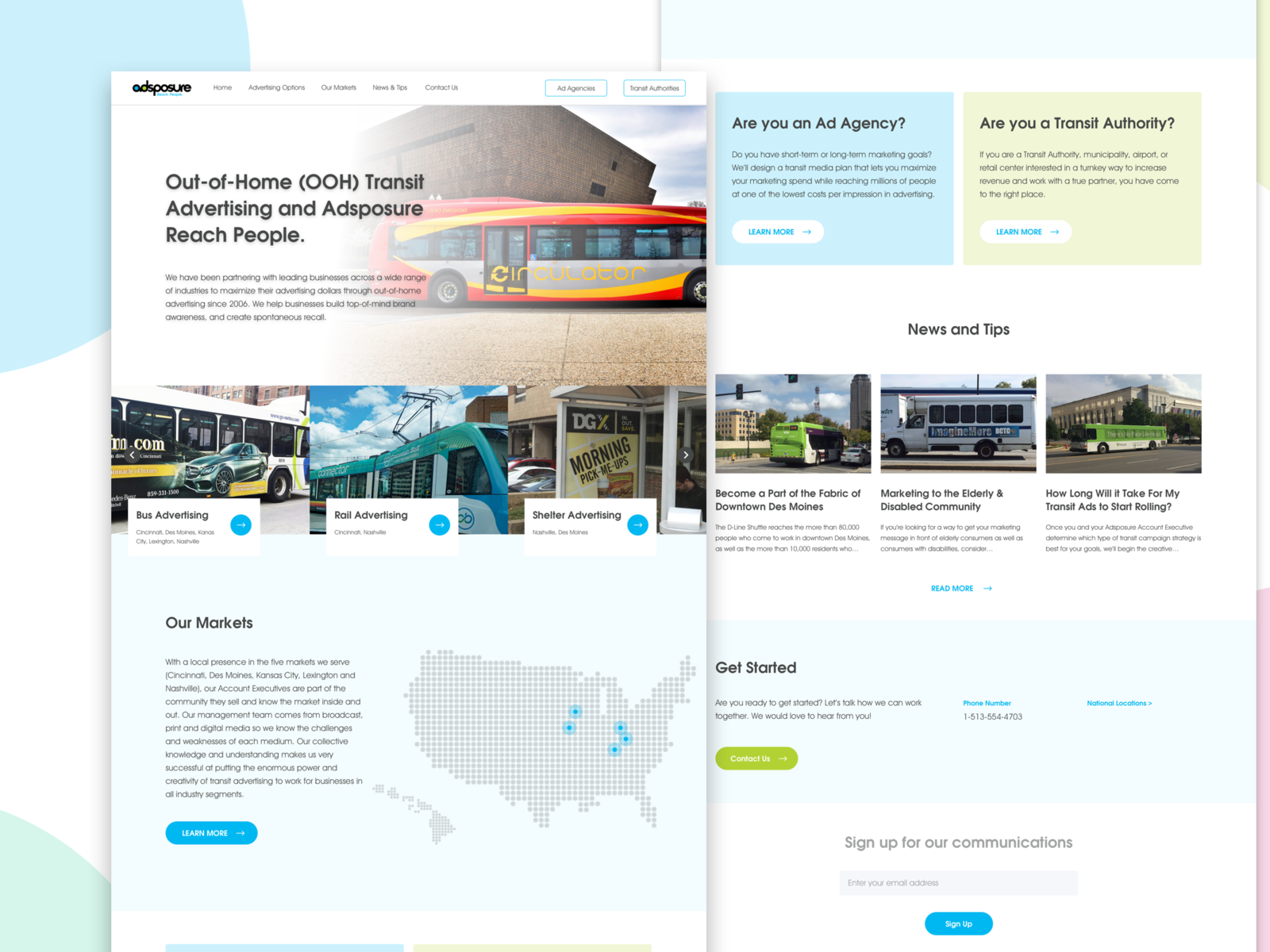This is a detailed mock-up of a dual-page web design featuring a white background with a subtle circle pattern. The pages are arranged side by side, with the left page slightly overlapping the right page.

On the top left corner of the left page, there's a header that includes the website's logo followed by five categorized links. Towards the right end of this header, there are two buttons outlined in light blue with white interiors containing text.

Beneath the header, a prominent photograph of a bus is displayed. To its left, there is a header text and a descriptive body of text beneath it. Below this section, three images are aligned horizontally: the first image depicts a bus, the middle one shows a tram, and the third is of a bus station. Directly below these images lies a text box.

Further down, a large blue box takes up significant screen space containing a headline that reads "Our Markets," followed by a body of text and another blue button. Adjacent to this, on the right, there is a map of the United States composed of white dots, with certain central areas highlighted in blue.

On the right page, the top section features two colored boxes: one blue and one yellow. Below these, a section titled "News and Tips" includes three photographs, each accompanied by a headline and a brief description. At the very bottom of this page, a blue box with the text "Get Started" is displayed next to a green button. Finally, there is a sign-up section for communications, which includes an input field for an email address and a blue button.